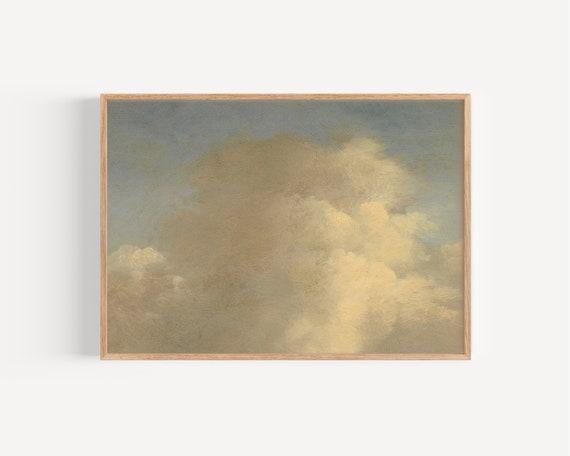This image depicts a framed painting with a brown wooden border. The painting is rectangular and showcases a sky and cloud scene. The sky occupies the upper portion of the painting and is painted in a blue hue. Below, various shades of cream, beige, and gray form a clump of clouds that extends slightly upwards in the middle and tapers downward on the sides. The background surrounding the painting is a light gray or cream color, providing a neutral contrast to the artwork. The cloud depiction is nuanced, incorporating gradients of dark and light cream, giving it an almost impure, textured appearance.